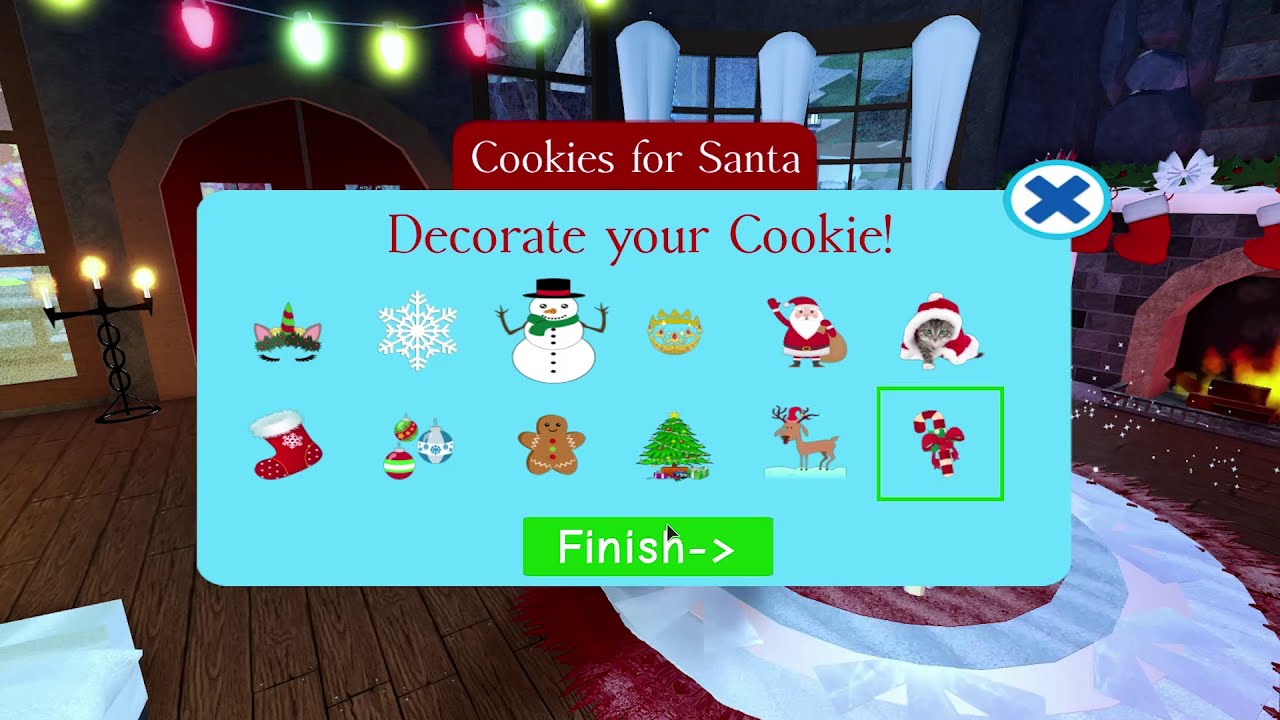The image appears to be a digital, animated scene likely from a Christmas-themed game or website. Dominating the foreground is a festive panel prompting the user to decorate a cookie for Santa, titled "Cookies for Santa" in white text on a red banner. Directly below, in a light blue rectangular box, instructions in red text read "Decorate your cookie." Arrays of selectable Christmas icons featuring characters and symbols such as a snowman, Santa Claus, a Christmas tree, candy canes, Rudolph, a snowflake, a gingerbread man, and a stocking are neatly organized in two rows of six icons each. At the bottom of this panel lies a green button labeled "Finish" in white text, indicating the final step in the cookie customization process.

The cozy, animated background depicts a warm Christmas living room. This room features wooden floors, a roaring fireplace adorned with stockings and flanked by candles in standing holders, a softly lit string of Christmas lights hanging above the door on the left, and a plush rug beneath. The inviting ambiance rounds out the scene, enhancing the festive spirit. It is evident that this detailed setup is intended to immerse the user in a joyful, interactive holiday experience.